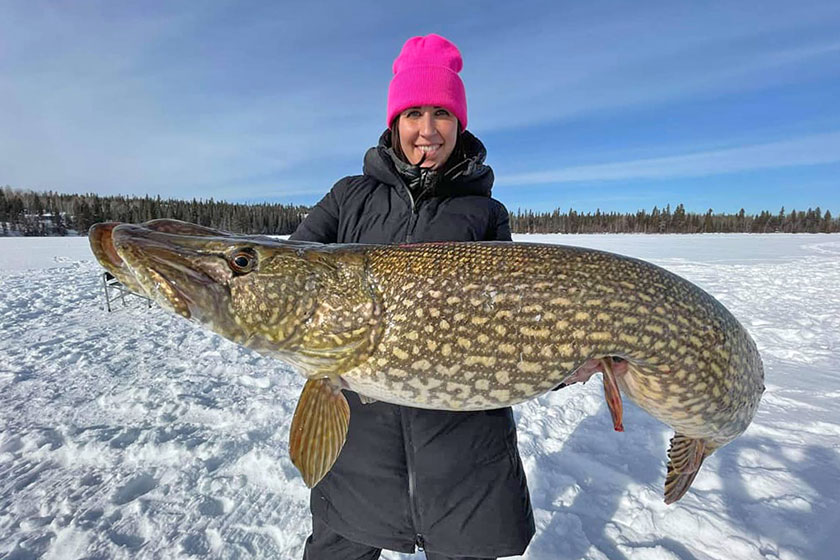The photograph features a horizontally oriented image showcasing a woman holding an impressively large fish that appears to be about six feet long. The fish, brown with beige speckles, curves with its tail positioned to the right side, bending slightly toward her. You can see its large eye and fins, with the woman’s hand supporting it from beneath, highlighting its immense size and weight. The woman is dressed warmly in a black puffy parka that reaches almost to her knees and a pink knit cap. She is smiling, revealing her top row of white teeth, and her dark hair frames her face. The background displays a snowy plain with numerous footprints and smooth patches of snow. In the distance, there's a row of pine trees and possibly a house to the left. The sky above is blue with a light overcast towards the left side, indicating a sunny day as suggested by the shadows cast behind the woman and the fish, including the shadow of the person taking the photograph visible at the bottom right.